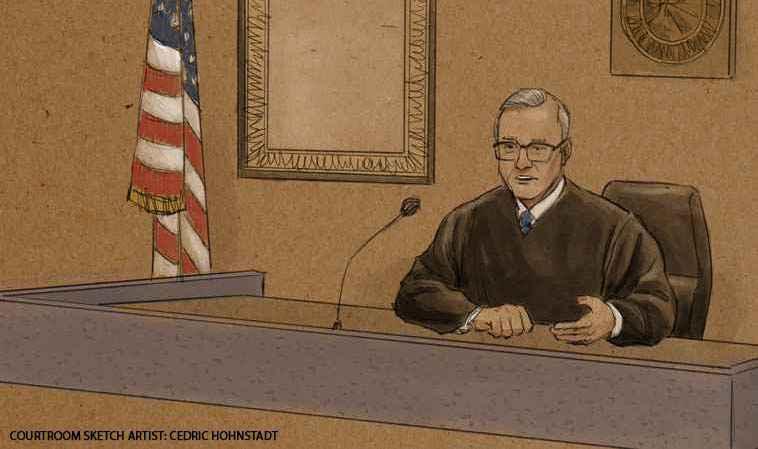This image is a colorful courtroom sketch by artist Cedric Hanstad. It depicts a judge with gray hair and square reading glasses, dressed in a black robe, with a blue tie partially visible underneath. The judge sits in a black leather chair behind a brown judge's bench, speaking into a microphone. The background features a brown-painted wall with a framed mirror and an American flag with red, white, and blue stripes to the judge's left. A clock is positioned on the top right-hand side. At the very bottom left-hand corner of the sketch, the text reads "Courtroom sketch artist Cedric Hanstad."